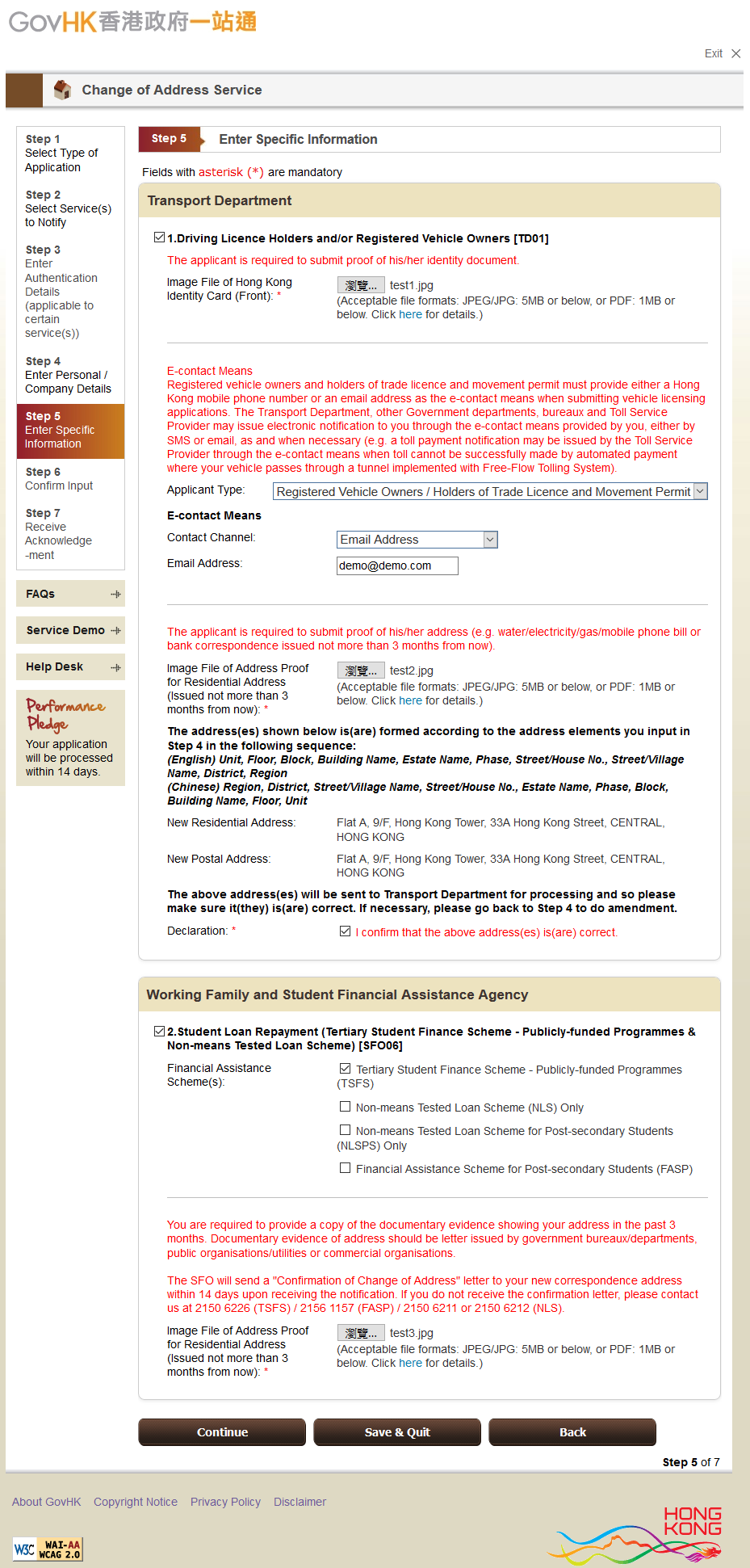This is a screenshot capturing the interface of a Chinese-language website, which seems to be optimized for either mobile or desktop viewing, though the exact platform isn't clear. In the upper left-hand corner, there is the text "gov HK," indicating that it is a government site for Hong Kong, followed by Chinese characters. Below this header, there is a prominently displayed horizontal bar labeled "Change of Address Service." The screenshot presents a lengthy webpage filled with numerous menus and items with relatively small, unreadable text, many of which are highlighted in red. Additionally, the words "Transport Department" are visible, suggesting that this website is related to the transportation department services in Hong Kong.